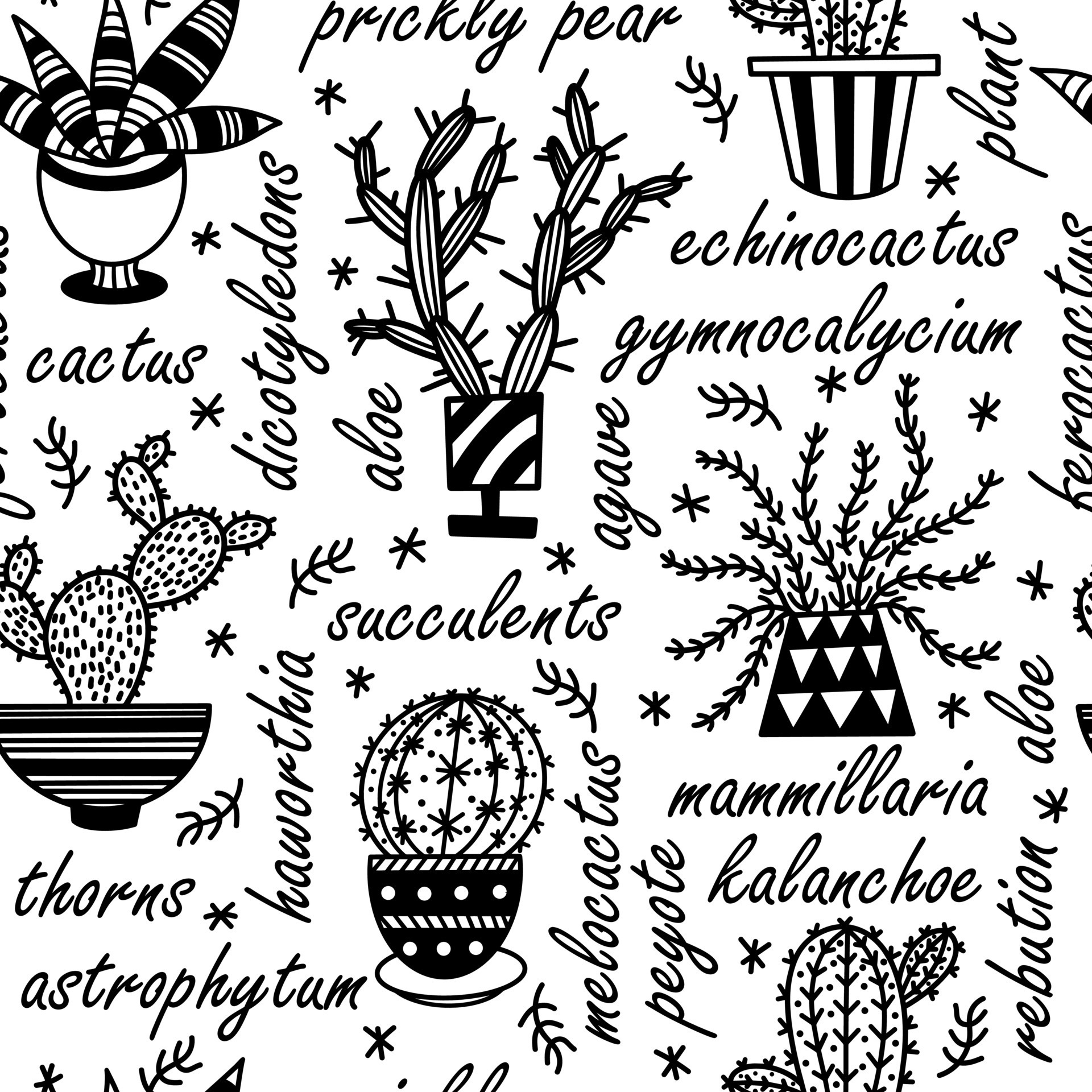This black and white graphic illustration resembles a hand-drawn pattern that might appear on fabric or wallpaper. It showcases a variety of desert plants, including several types of cacti and succulents, each meticulously labeled with their scientific names in cursive writing. Positioned within decorative, folk-art-style containers, the plants include Cactus, Prickly Pear, Astrophytum, Aloe, Echinocactus, Gymnocalycium, and Mammillaria, among others. On the left side of the image, a prominent cactus appears, while the labels for other plants like Succulents, Thorns, and Kalanchoe are distributed throughout. Seven distinct plants are depicted in total, their varying shapes—from round with sharp points to the classic tall, segmented forms—highlighting the diversity of southwestern flora.